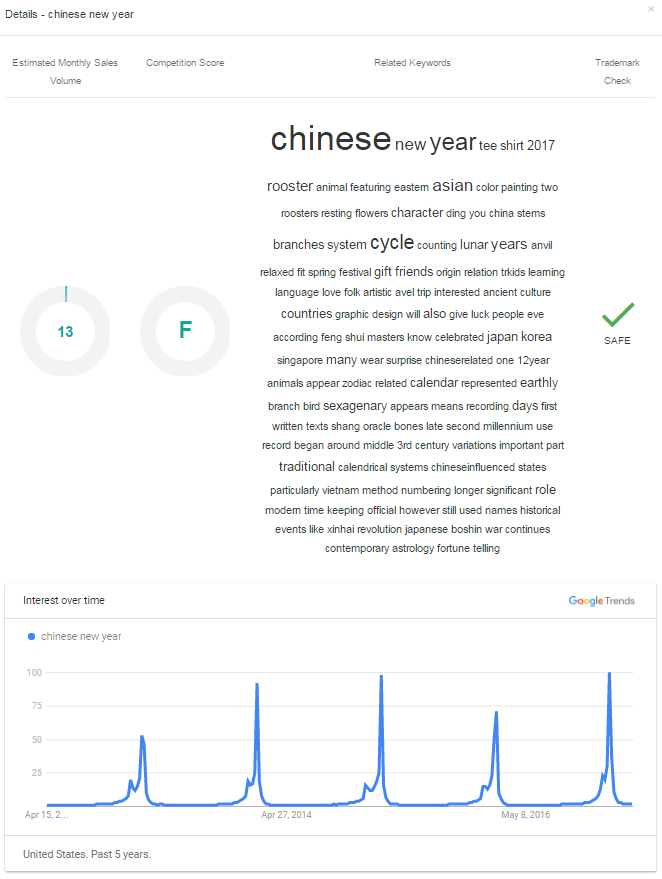In this image, we see a product listing screenshot set against a white background. In the upper left corner, it details "Chinese New Year." Below that, it includes sections for the estimated monthly sales volume, competition score, and related keywords. The product in focus is a "Chinese New Year T-shirt 2017" featuring a rooster, an important symbol in Eastern Asian culture, depicted through color painting.

The design showcases two roosters resting amidst floral arrangements, with characters and motifs from traditional Ding Yu China. Branches signify the cycle and system of counting lunar years. The T-shirt boasts a relaxed fit, making it perfect for the Spring Festival. 

It is an ideal gift for friends and is rich in cultural significance. This product connects to themes of origin, relationships, language learning, love, and folk art. It offers a graphic design that is not only visually appealing but also intended to bring good luck according to Feng Shui principles. Chinese New Year is celebrated in several countries, including Japan, Korea, and Singapore, highlighting its broad cultural impact and significance.